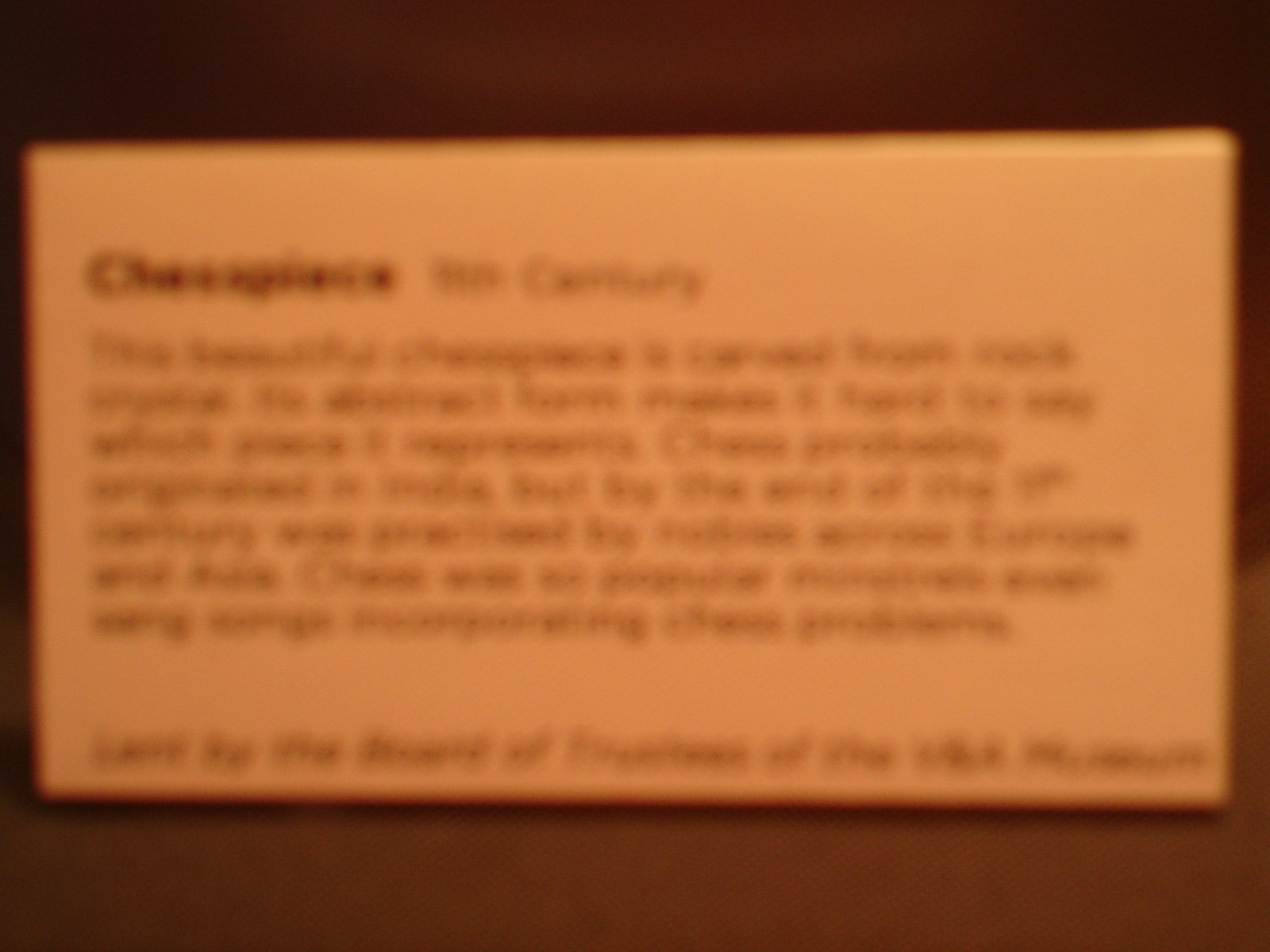The image features a highly blurry photograph of an art installation or museum piece descriptor plaque. Typically, these plaques are white and small, located at the bottom or side of the art piece. However, this particular plaque is illuminated by an orange light, causing the plaque itself to appear in a lighter shade of orange against a darker orange background. The text is completely unreadable due to the blurriness, but the layout is discernible: the title at the top left in bold, followed by seven lines of regular text beneath it, and a single line of text separated from the paragraph at the very bottom. Shadows flank the plaque on both sides. Despite the overall lack of clarity, there is a small possibility that one of the words in the top line could be "century." The text appears to be written in black ink.